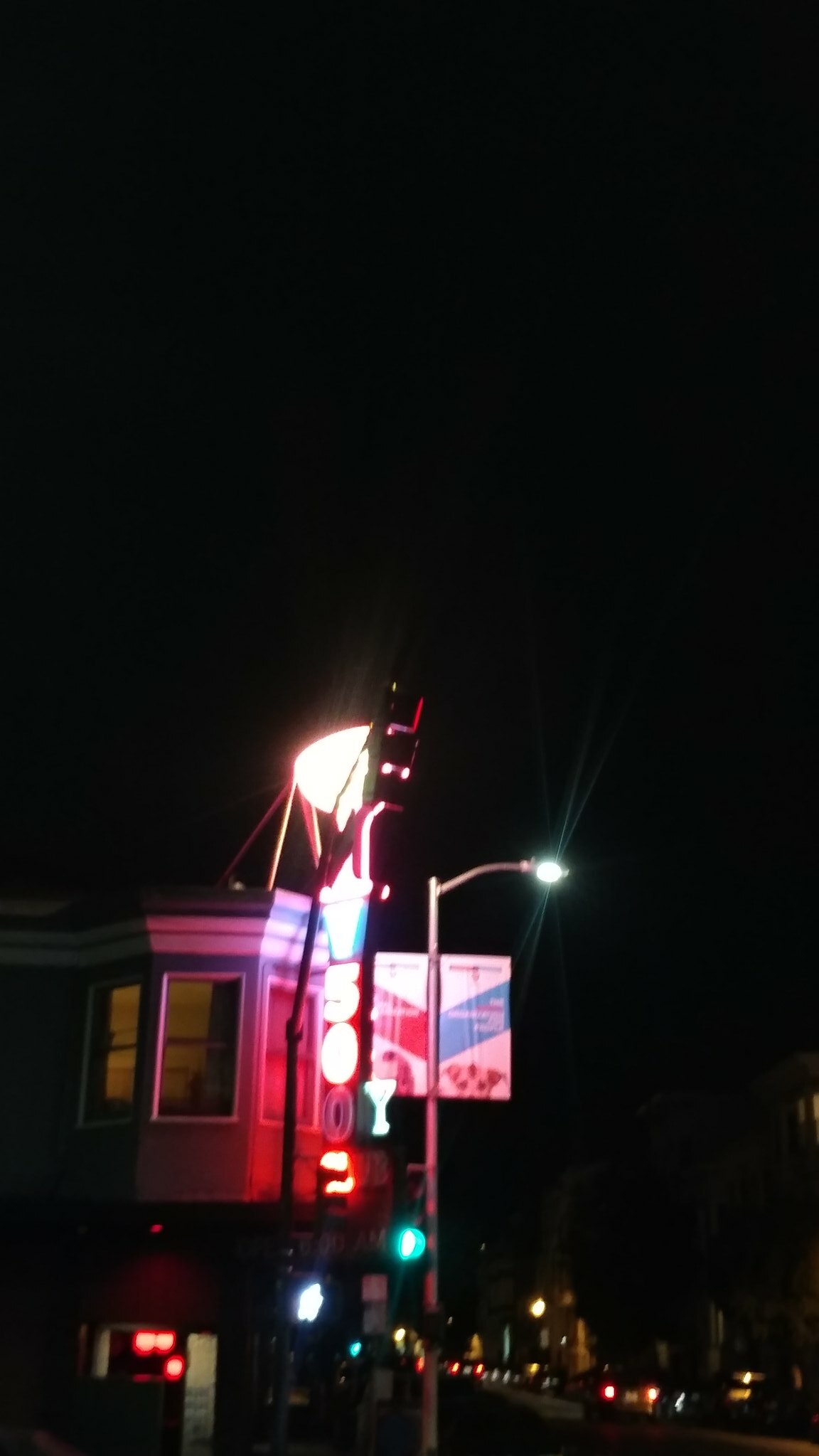This nighttime cityscape captures a scene bathed in darkness, punctuated by various lights. Dominating the foreground is a streetlight pole standing centrally, topped with a bright lamp that casts a glow onto the surroundings. Adjacent to this pole is a functional green traffic light, adding a pop of color to the monochromatic backdrop.

In the distance, nestled in the lower right-hand corner, a constellation of lights marks the presence of small buildings and what appear to be car taillights, hinting at a road or boulevard.

Midway up the image, a dome-shaped, large white light commands attention. To its side, another traffic light stands, adding to the urban infrastructure. Below this, a neon sign declares "V500," although the rightmost zero is dimmed, no longer illuminating as intended.

This neon sign is affixed to a two-story building, whose architecture reveals an octagonal facade on the upper level with three visible windows. The ground floor presents a more straightforward design with a white door centrally located, possibly functioning as an entryway to a shop or dwelling. The overall composition, with its interplay of artificial lights and architectural elements against the nocturnal void, imparts a tranquil yet vibrant urban feel.